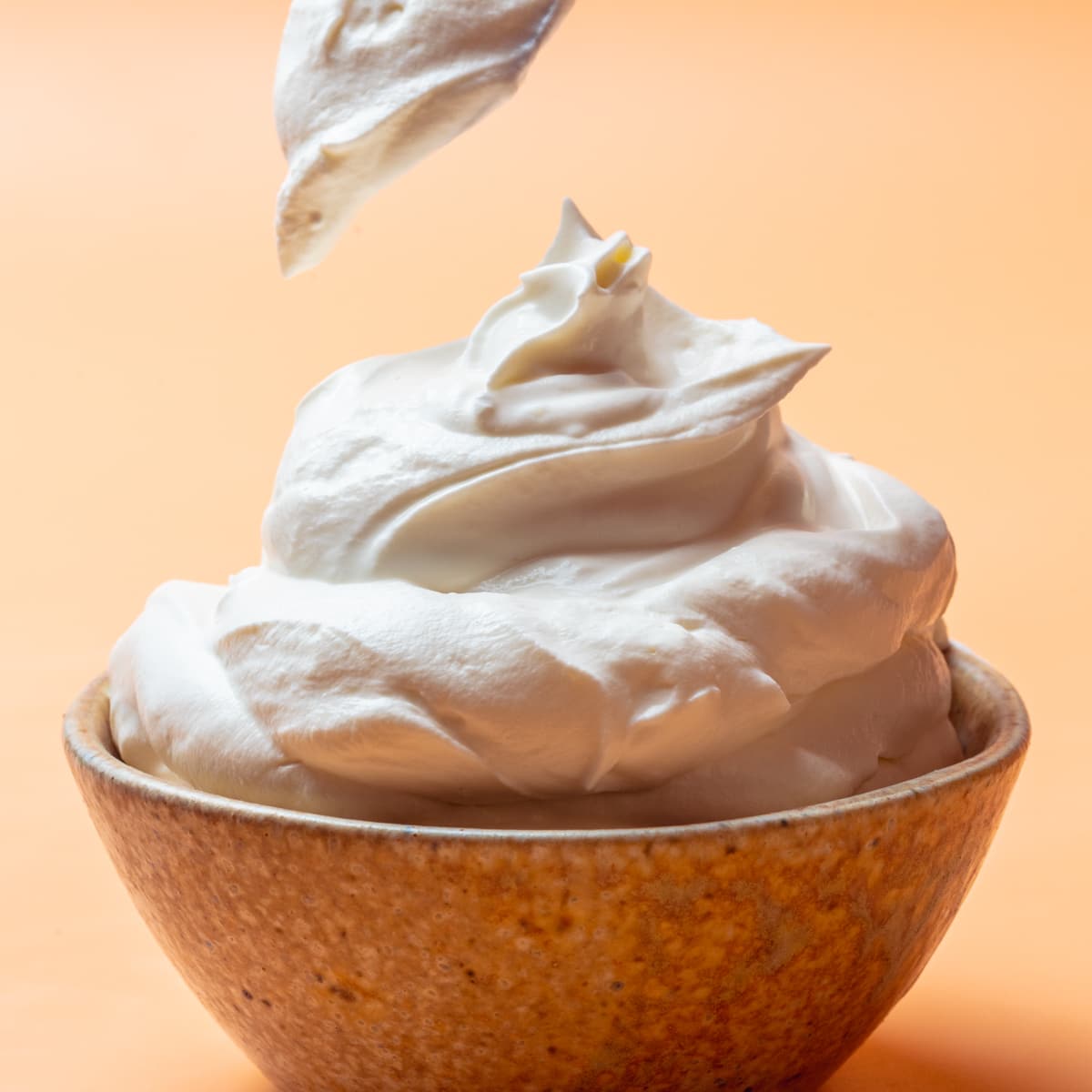The photograph features a central stone-like beige-brown bowl set against a gradient peach-orange background that is darker at the top-right corner and gradually lightens throughout, except for the bottom right where a shadow makes the peach color subtly darker. The bowl is filled with what appears to be soft serve ice cream or vegan whipped cream. The creamy, off-white substance is mounded high above the rim of the bowl, forming soft peaks that suggest a fluffy and airy texture. There's a spoon descending from the top middle of the image, with a small amount of this soft, light brown-ish cream starting to fall off its back. The overall composition highlights the creamy texture and the inviting swirl formations within the bowl.